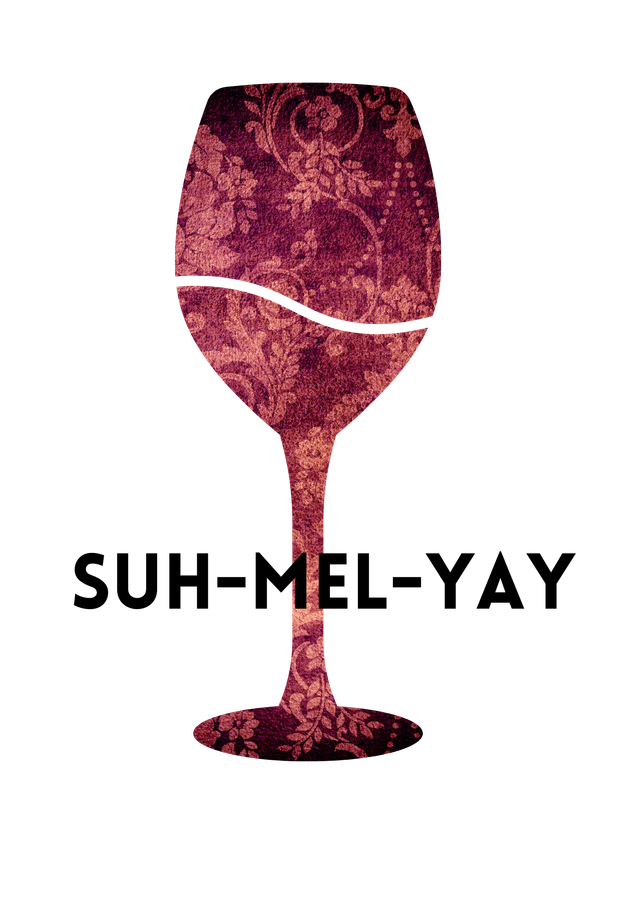The image features an abstract silhouette of a wine glass set against a plain white background, occupying the central space and reaching about three to four inches high. The wine glass is not realistic but rather an outline adorned with a textured fabric pattern reminiscent of a fuzzy blanket often seen on a grandma's couch. The fabric displays a rich burgundy color with intricate floral patterns in shades of orange, pink, and beige, complete with delicate vines and leaves. In the upper portion of the glass, a white, wavy line traverses from left to right, slightly higher on the left and sloping downwards to the right. At the bottom part of the stem, in bold, all-uppercase black letters, the text "S-U-H-M-E-L-Y-A-Y" is prominently displayed.